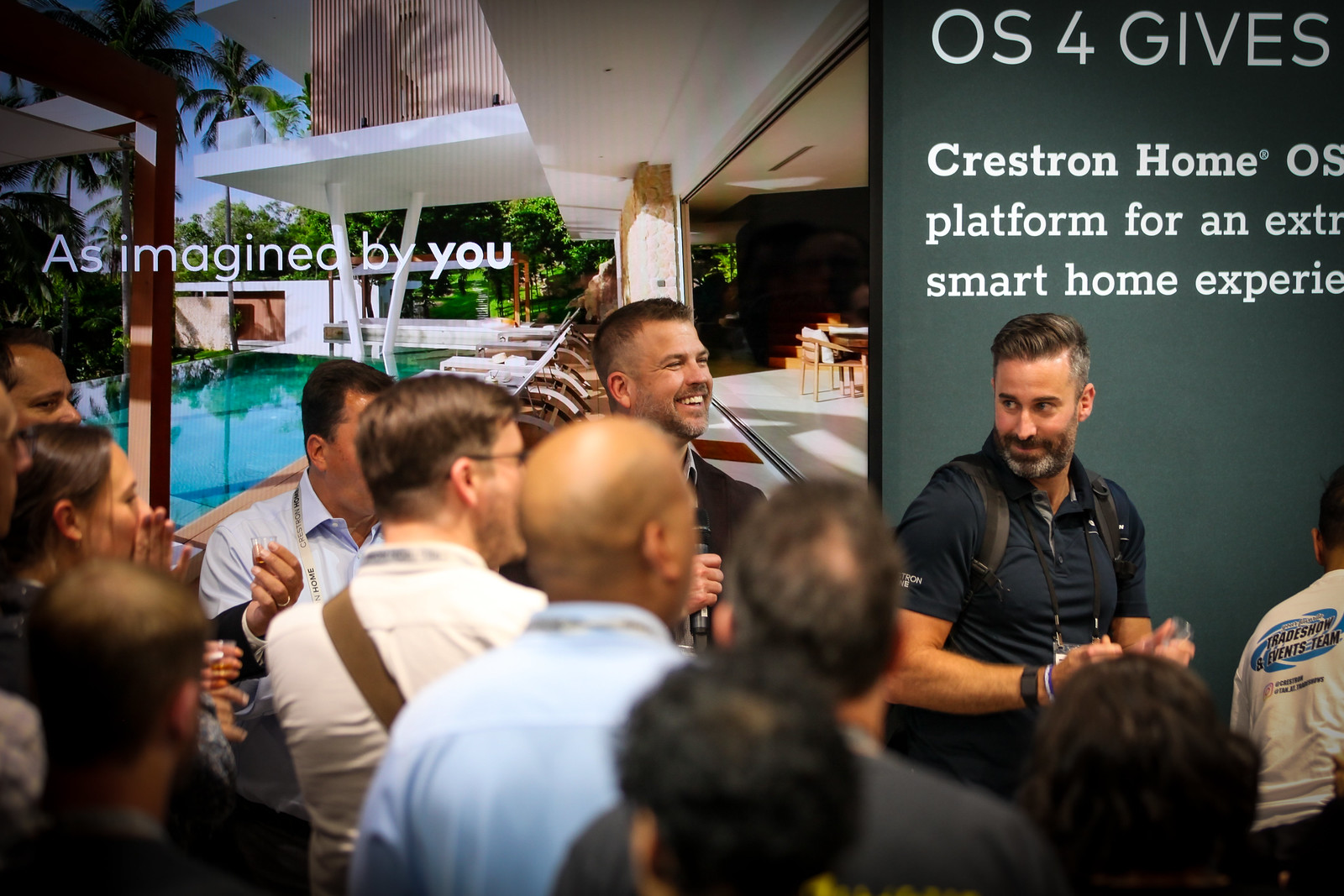This horizontal rectangular image appears to be an advertisement for a company named OS4, promoting the Crestron Home Platform for an advanced smart home experience. The right side of the image features a forest green panel with white text that reads "OS4 gives Crestron Home Platform for an extra smart home experience." Below this text, a man with salt-and-pepper hair and a brown beard, dressed in a dark navy shirt, sits smiling. He faces a large crowd on the left side of the image, which consists mostly of men with a few women, all smiling and looking toward him. This crowd is standing in front of the scene that depicts a modern, luxurious home environment with a pool, a large deck, and several patio chairs, indicating a high-end, possibly tropical setting. Across this background image, the phrase "as imagined by you" is boldly superimposed in white letters. The scene suggests a professional event, possibly a trade show or presentation, with the ambiance resembling that of a resort or upscale residential setting.